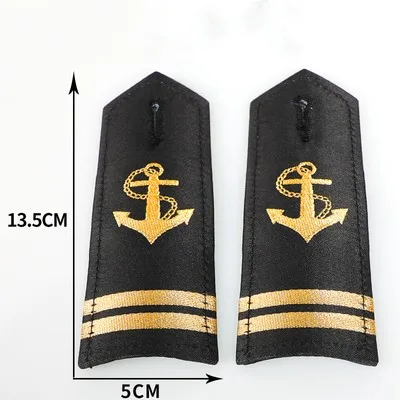This isolated photograph shows two identical naval epaulets, often worn on the shoulders of military or naval officers. Each epaulet measures 13.5 centimeters in length and 5 centimeters in width. The rectangular-shaped epaulets are black with a triangular, pointed top that features a buttonhole for attachment to a uniform. The centerpiece of each epaulet is a gold anchor with an interwoven gold chain, facing downwards. At the bottom of each epaulet, there are two horizontal gold bars, indicative of a lieutenant's rank. Both epaulets are bordered with black stitching and are positioned vertically side-by-side against a dark navy blue background. The measurement indicators, "13.5 CM" and "5 CM," are marked on the left and bottom of the image, respectively, and the entire setup is displayed against a clean white backdrop.